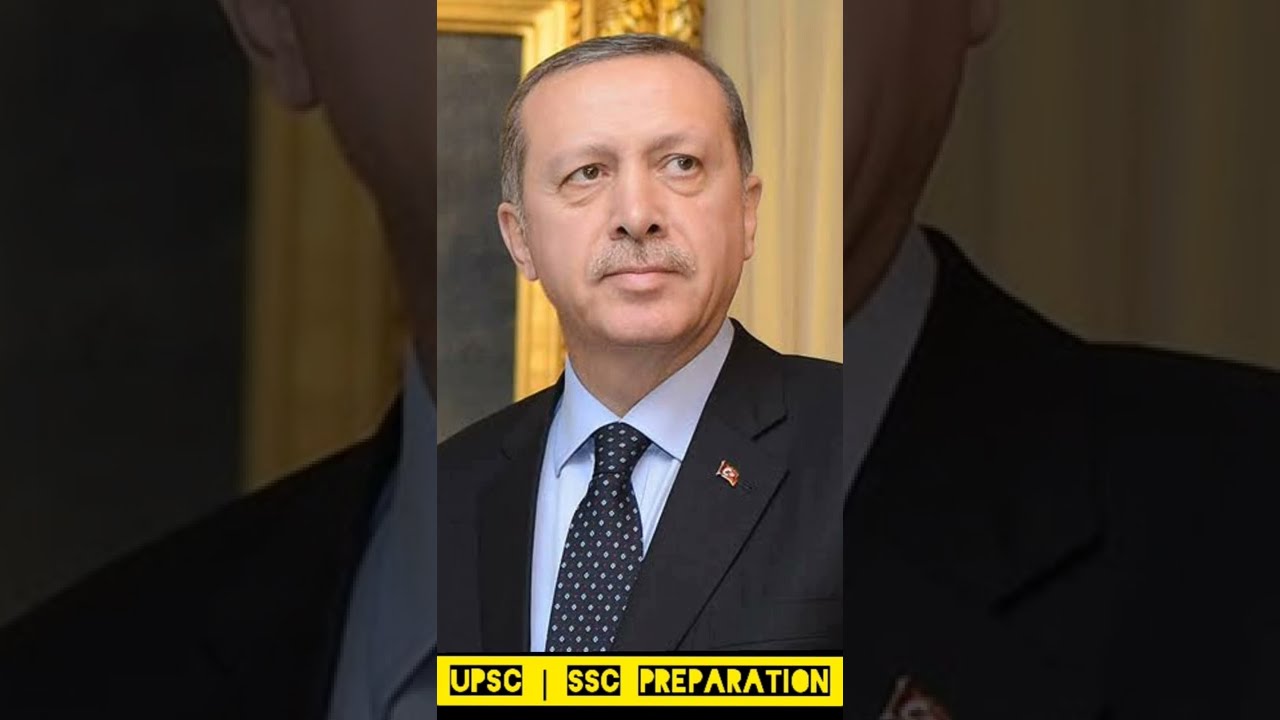The image is a detailed close-up headshot of a middle-aged to late-50s man with salt-and-pepper, receding hair and a thin mustache. He has dark eyes looking off to the left side of the image. He is dressed in a black suit with a light blue button-down shirt, and a navy blue tie featuring some form of dot or checkered design. A small, indistinctive pin is visible on one side of his jacket. Behind him, there is a large gold frame partially visible, indicating it might be the edge of a picture or mirror but cut off from the view. The background features a distinct yellow rectangle at the bottom of the image, displaying the text “UPSC SSC preparation” with the letters having a black outline. The golden frame and the specific text in the yellow background highlight the context of the image, suggesting it ties to exam preparation visuals.